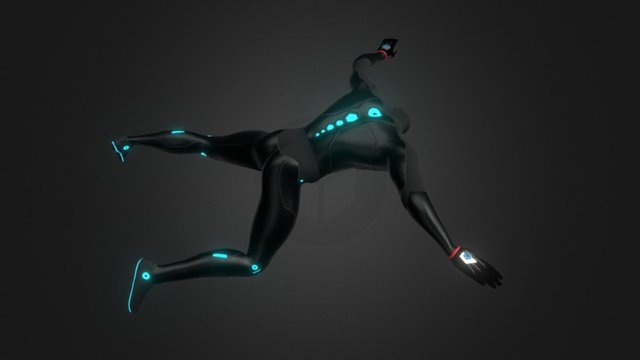This digital art piece presents a computer-generated humanoid figure suspended in a horizontal, rectangular frame with a gradient background transitioning from black at the edges to a lighter gray in the center. The humanoid, lacking a head, appears to be in a state of free fall with its arms and legs outstretched. The entire body is predominantly black, resembling an advanced cybernetic or robotic form clad in a sleek bodysuit. Intricately detailed with glowing blue LEDs, the figure features a series of turquoise points along the spine, at the knees, ankles, and the underside of the feet. These LEDs create a striking contrast against the dark figure. Additionally, the figure's wrists are accented with red wristbands. The arms are adorned with what seem to be black gloves highlighted by glowing white sections. The overall aesthetic aligns with a cyberpunk theme, giving the figure a futuristic and enigmatic appearance as it floats, appearing to fall through space.